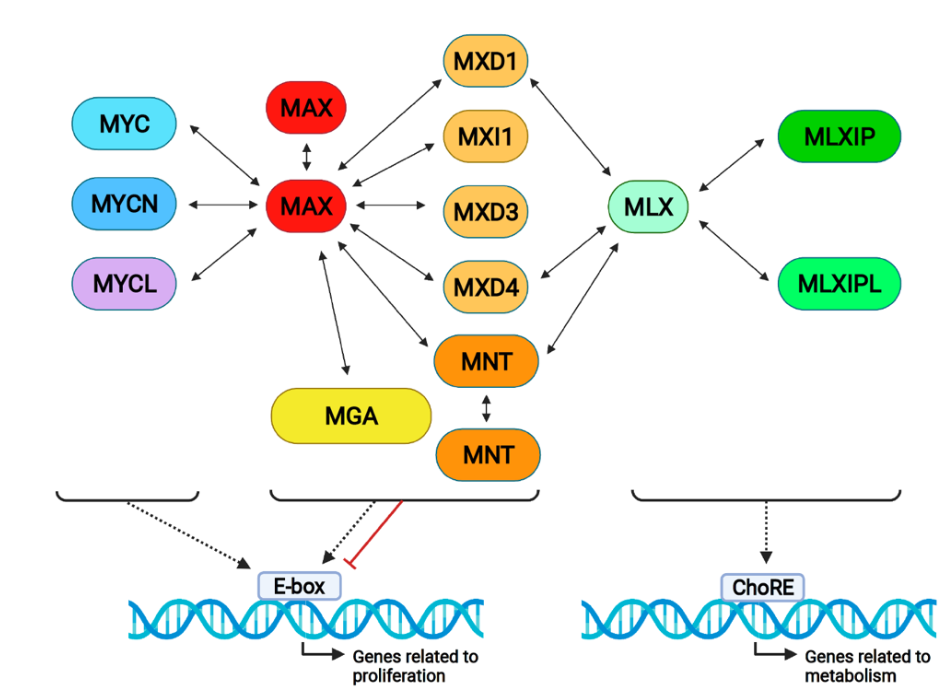This is a detailed diagram depicting various interactions among chemical compounds, likely related to medical or biochemical processes. The image features numerous pill-shaped colored ovals, each labeled with acronyms such as MYC, MYCN, MYCL in blue and purple on the left, and MGA, MNT, MXD4, MXD3, MXI1, MXD1 in shades of yellow, orange, and green on the right. Two red ovals labeled MAX are centrally positioned, linking multiple interactions. A light green oval is labeled MLX, with slightly darker green ovals marked as MLXIP and MLXIPL. 

Towards the bottom, a rectangular box labeled "EBOX, genes related to proliferation" indicates the role of the orange, red, and blue ovals. Additionally, wavy blue lines and black arrows illustrate the relationships and interactions between these various compounds. Text throughout the diagram is in black, ensuring clarity in detailing these complex biochemical relationships.